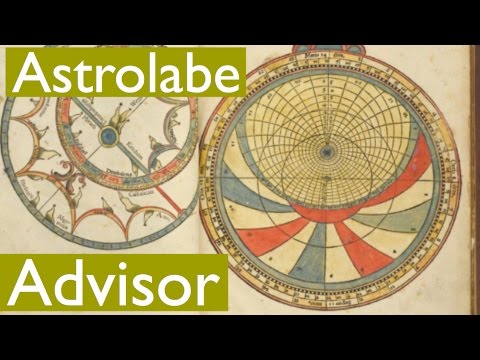The poster titled "Astrolabe Advisor" features a vintage aesthetic with a dominant beige-yellow background. Centered on the poster are two intricately designed, circular astrolabes, one on the left and one on the right. Each astrolabe showcases elaborate markings and designs, reminiscent of ancient astronomical instruments. The astrolabe on the left has a dark gray border with sunbeam-like, pointed maroon extensions inside, forming a semi-circle with deep blue accents at its core. The right astrolabe is outlined in gold and displays a dynamic combination of blue, white, and red, arranged in a pinwheel fashion, interspersed with potential numbers and letters. The top left corner of the poster prominently displays the word "Astrolabe" in white lettering against a green background, while the bottom left corner features the word "Advisor" in white, unifying the theme of ancient celestial navigation instruments.